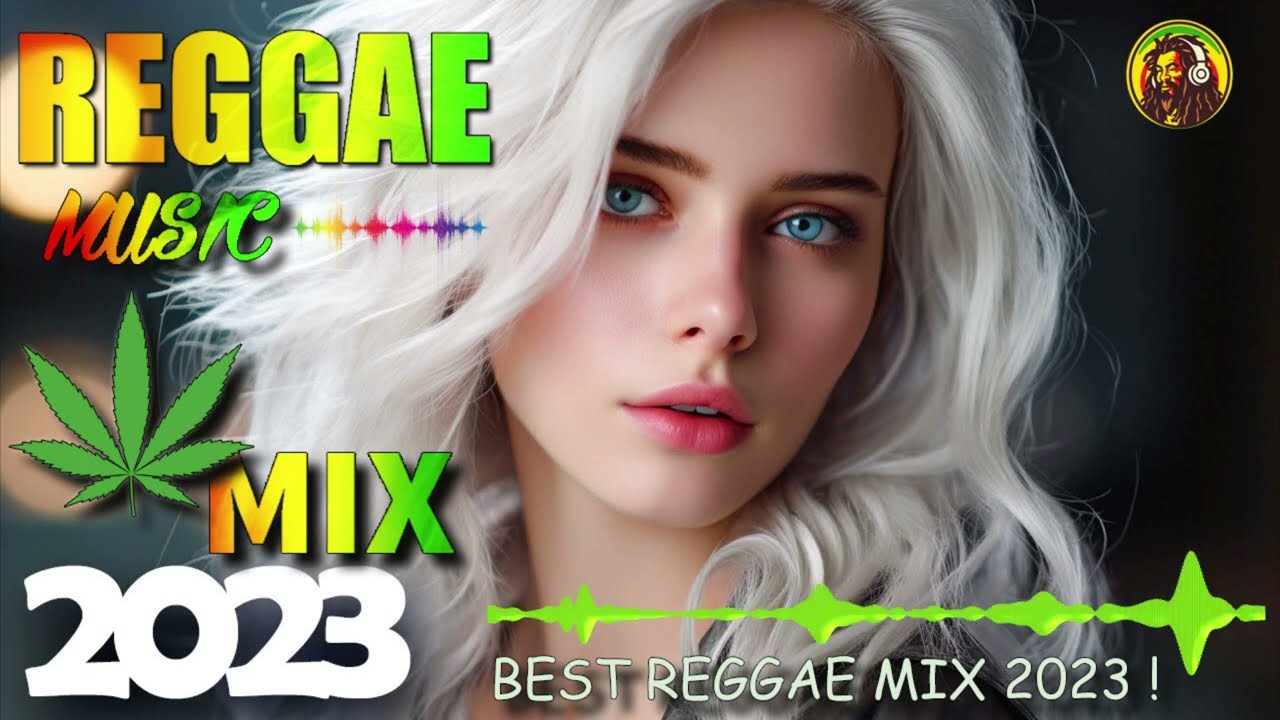This wide rectangular digital advertisement features a highly realistic depiction of a young white woman with striking bright blue eyes, brown eyebrows, and slightly open pink lips, her expression imbued with a hint of seduction. Her long, thick, wavy hair is a striking silver or white. The image is intimately cropped to focus on her face, cutting off just below her neck, with no visible clothing.

In the top left corner, vibrant text in red, yellow, and green gradient reads: "Reggae Music Mix 2023," with a white "2023" and a marijuana leaf placed prominently before the word "Mix." On the bottom right, similar text declares: "Best Reggae Mix 2023." The advertisement is completed with a logo in the top right corner, depicting a Rastafarian man with dreadlocks wearing white over-ear headphones. The upper right corner also features green sound wave graphics, adding a dynamic touch to the overall design.